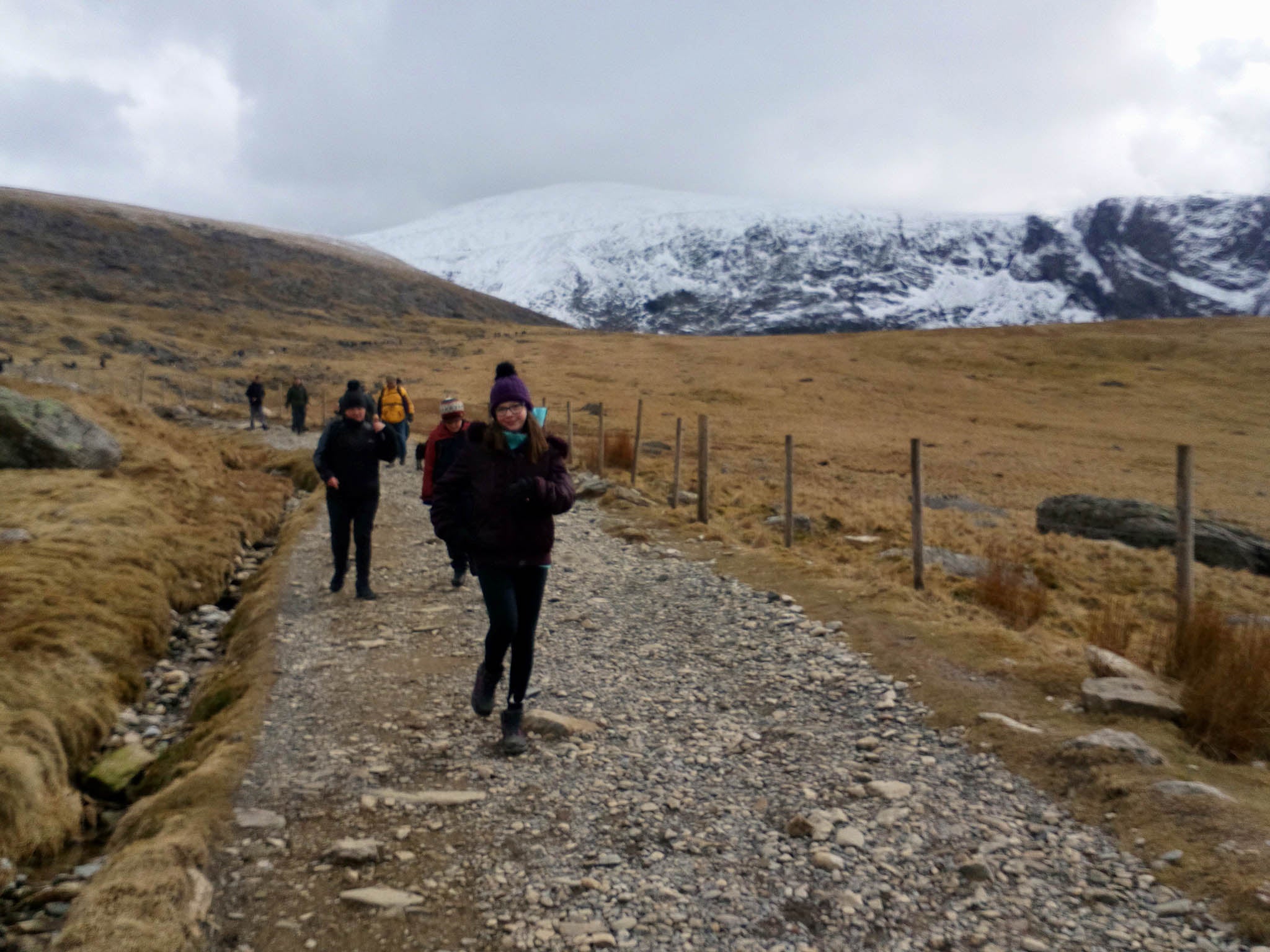In this image, a group of six people is seen hiking along a stony path that extends from the forefront center and angles slightly to the left as it recedes into the distance. They are all donned in jackets, hats, and a variety of long pants, indicating the cold weather. The pathway is flanked by fields on both sides, with a small trench or ditch on the left and a row of posts, likely meant for a fence, on the right. The landscape appears relatively barren with rocks and logs but scarce in trees. In the background, the scene features a brown hill to the left and snow-covered mountains in the far distance to the right, beneath a gray, cloudy sky. A notable feature includes a smiling girl in a purple hat and jacket leading the group, who are all moving in the same direction. Patches of evergreen trees can be seen on the distant mountain ridges, amidst a primarily wheat-burnt orange grassy field. To the left of the path stands a large gray rock, with a flat dark-colored rock on the right.